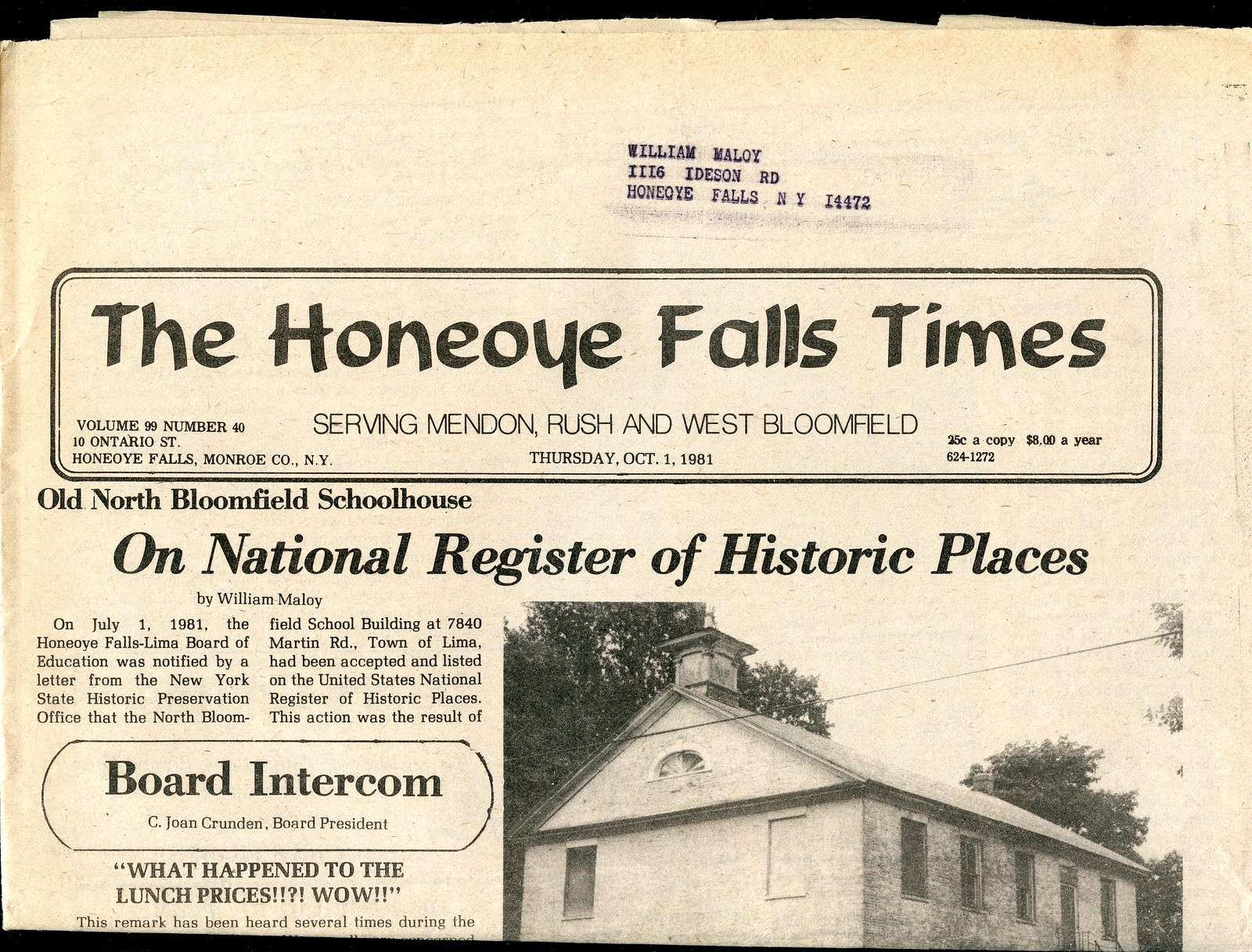A black-and-white image of an aged, cream-colored newspaper front features a clipping from "The Honeoye Falls Times," dated Thursday, October 1st, 1981. Addressed to William Malloy at 1116 Ideson Road, Honeoye Falls, NY, 14472, the newspaper headline reads, "The Honeoye Falls Times, Serving Minden, Rush, and West Bloomfield." Prominently, there is an article titled "Old North Bloomfield Schoolhouse on National Register of Historic Places." This article, written by William Malloy, announces that on July 1st, 1981, the Honeoye Falls Lima Board of Education received a letter from the New York State Historic Preservation Office, confirming the listing of the North Bloomfield School Building at 7840 Martin Road, Town of Lima, on the United States National Register of Historic Places. The front page also includes a black and white photograph of the schoolhouse, showing its four-windowed side, a chimney on top, and trees in the background. Additionally, an adjacent article, partially visible, intriguingly questions, "What happened to the lunch prices?"